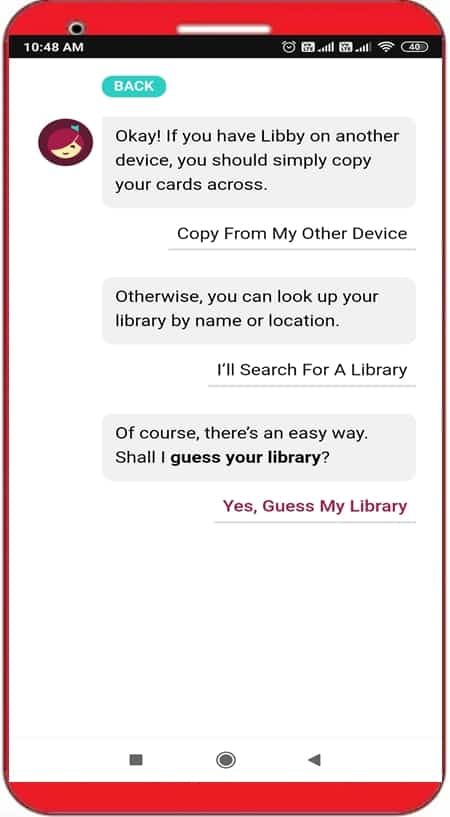The screenshot depicts a conversation on a mobile device with red borders indicating the edges of the smartphone. At the top border, there's a thin black bar displaying typical mobile interface icons. On the left corner, the time reads 10:48 a.m. To the right are various status icons, including an alarm clock, square icons, a Wi-Fi signal indicator, and a battery icon showing 40% charge.

Below this, the main screen features a white background. At the top left, a turquoise oval button marked “BACK” in white letters stands out. The conversation between two people is laid out beneath this button.

The first message on the screen, originating from the left, is indicated by a circular avatar. This avatar showcases a cartoon-styled girl's head with reddish-purple hair falling over one eye, a small smile, and has a brown background. The accompanying message is in a light gray speech bubble and reads, "OK! If you have Libby on another device, you should simply copy your cards across."

The next message, from the right side, appears in a white speech bubble, partially outlined, stating, "Copy from my other device."

Another message from the left side in a gray speech bubble follows, "Otherwise, you can look up your library by name or location." Subsequently, a response from the right side in a white speech bubble reads, "I'll search for a library."

Further down, a gray speech bubble from the left says, "Of course, there's an easy way, shall I guess your library?" The final visible message, coming from the right in a white speech bubble with a dark purplish-brownish font, says, "Yes, guess my library."

At the bottom of the screen, a navigation bar displays three buttons commonly found on mobile devices: a gray square button on the left, a circular button in the middle, and a sideways triangle (with the point facing left) on the right. The rest of the space appears blank, indicating the end of this segment of the conversation.